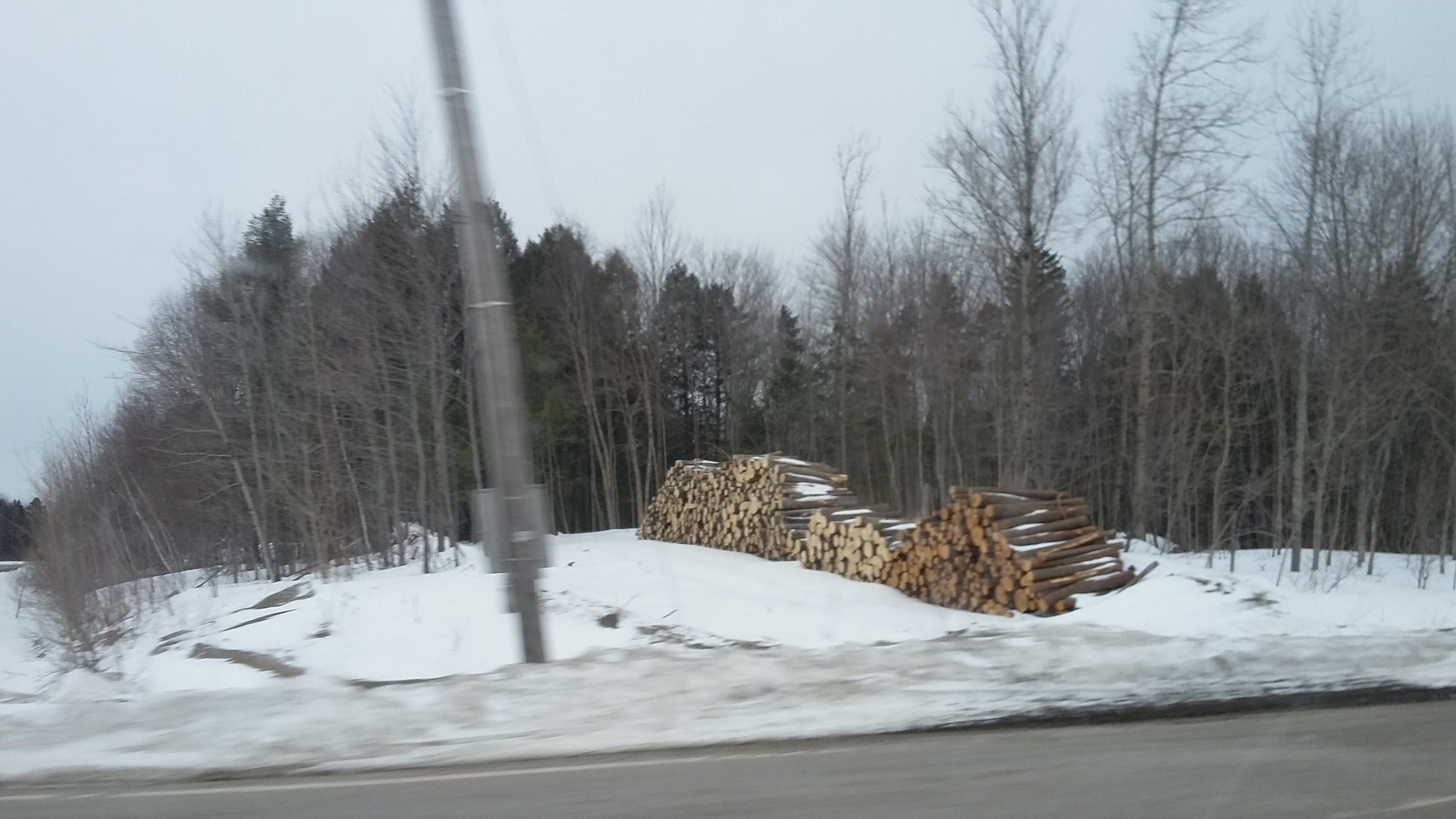The image captures a snowy field layered with intricate details. In the foreground, the bottom section reveals a snow-free road made of black asphalt, bordered by some blurred concrete elements and perhaps wooden separators. Approximately 20% to the left of center, a blurred pole stands next to the road. The middle ground showcases a vast white snowy field, interrupted by a large, neatly stacked pile of firewood composed of varying hues: dark brown, lighter tan, and a greenish-brown, each log appearing to come from different parts of trees. There seem to be over 100 logs, hinting at a substantial stockpile. Deciduous trees, stripped bare by winter, are scattered in the foreground, contrasting with the darker presence of pine or cedar trees in the background, which create a dense, shadowed area. The sky above is overcast and gray, adding to the wintry ambiance of the scene.